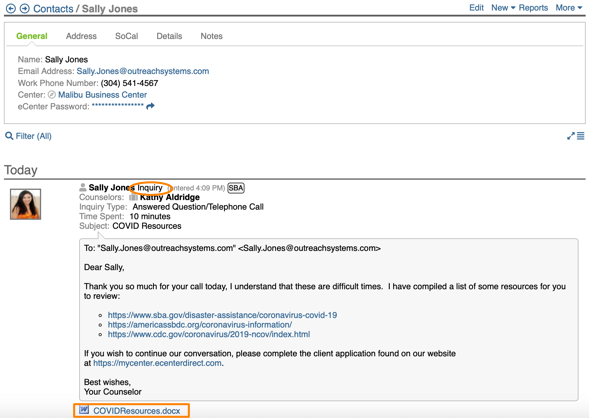The image shows a highly magnified section of an email, specifically zoomed in to 200%. At the top of the email, there is a section labeled "Contacts" featuring the information for Sally Jones. The general details listed are as follows:

- **Name:** Sally Jones
- **Email Address:** outreachsystems.com (highlighted in blue)
- **Work Phone:** 304-541-4567
- **Center:** Malibu Business Center

Additionally, there is a section with the eCenter password that is crossed out with decorative symbols resembling small flowers. 

The email was sent today, and next to the date, there is a small thumbnail picture of Sally. The subject line of the email is "COVID Resources."

The content of the email includes information on various counselors, mentioning in particular Kathy Aldridge, and flagged as an "Inquiry Type: Answered Questions" from a "Telephone Call." It also notes that the counselor spent 10 minutes on the inquiry.

The email, addressed to Sally from her counselor, reads:
"Dear Sally,
Thank you so much for your call today. I understand that these are difficult times. I've compiled a list of some resources for you to review."

This detailed description encapsulates the visual and textual elements present in the magnified email image.